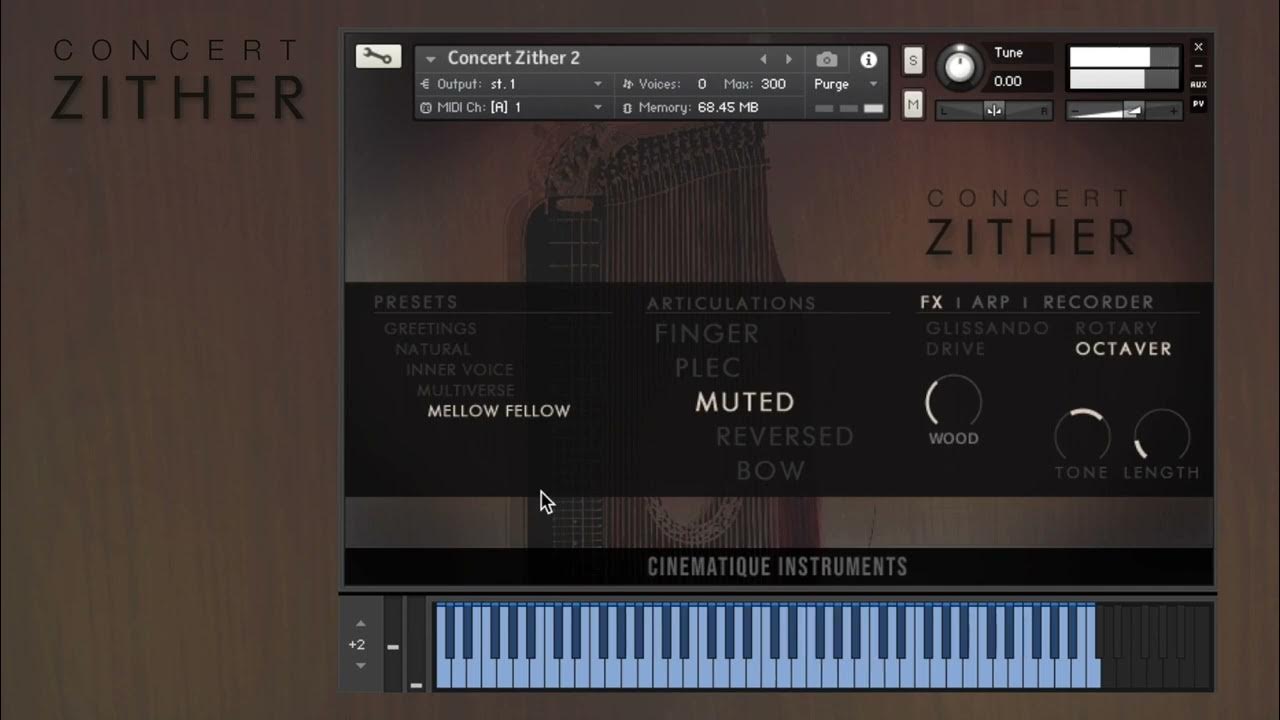The image is a detailed screenshot of a digital music orchestrator or mixer interface, labeled "Concert Zither". The centerpiece of the interface features a digital piano keyboard stretching across the bottom. On the left side of the keyboard, there are adjustable sliders with up-and-down indicators currently set to plus two. Above this, a smaller inset image displays the current presets chosen by the creator. The top of the interface contains a tool bar listing various options such as the output, channels, voice, memory, and tuning capabilities.

Prominently displayed in the middle are preset options listed as "Greetings," "Natural," "Inner Voice," "Multiverse," with the current setting highlighted in white as "Mellow Fellow." Directly below this, there are articulation options including "Finger," "Plec," "Muted," "Reversed," and "Bow," with "Muted" shown in white.

On the right-hand side, additional settings are available for "Wood" and "Octaver," where various tone and length settings have been selected. The bottom right corner is marked with “Cinematic Instruments” against a black bar background. The complex interface includes numerous details and smaller text that is difficult to read, but it combines elements of a zither instrument and electronic music production tools, all presented in various shades of gray, white, and blue.